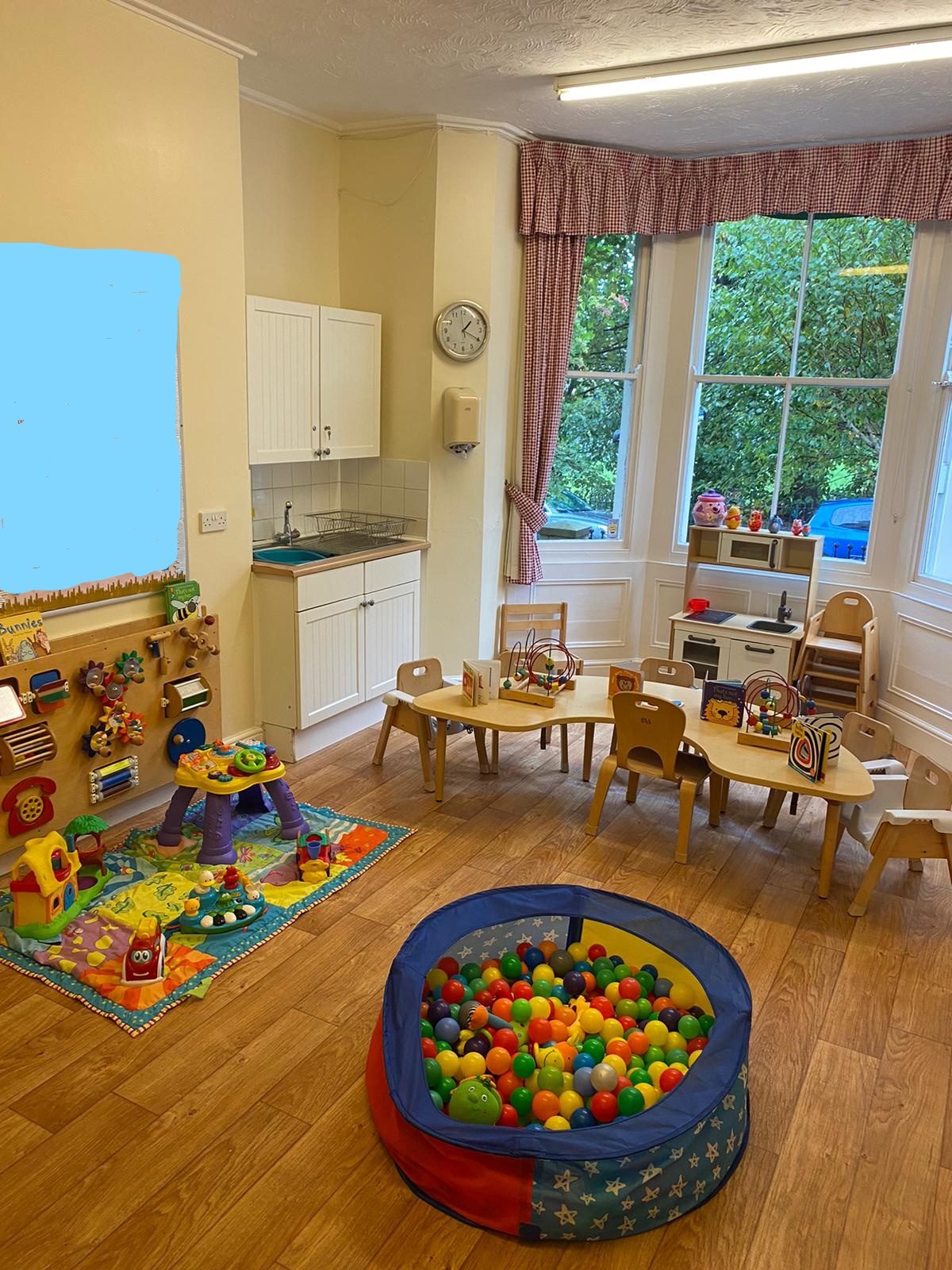This photograph captures a well-lit children's playroom inside a house, featuring a prominent bay window adorned with curtains held back on either side, revealing lush greenery outside. The room has wooden flooring and a colorful rug on which various toys are scattered. In the center, there's a soft, round container filled with numerous rubber balls for children to jump into and play. A small table, suitable for toddlers, is stocked with toys. On the right side, a board and additional toys are mounted on the wall, enhancing the playful atmosphere. In front of the bay window stands a miniature play kitchen, complete with a tiny sink and oven, perfect for imaginative play.